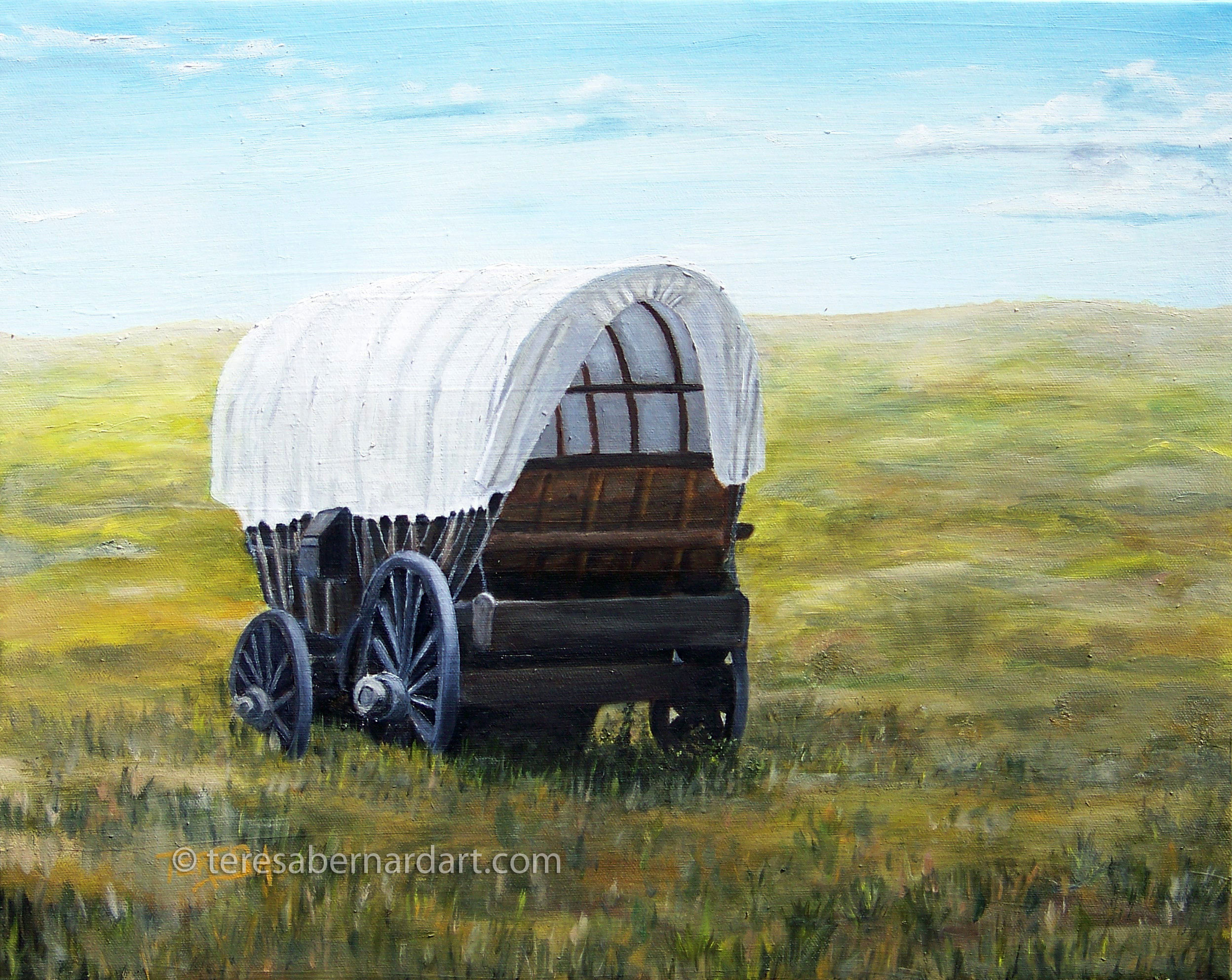The image is an oil painting depicting an abandoned covered wagon set in a hilly prairie field. The foreground showcases the wagon made of dark brown wood, with a white canvas canopy over it. The canvas, free from dirt or tears, is tied securely to the axles and supported by visible wooden ribs. The wagon is deserted, with an unoccupied front bench seat for the driver. One of its large, gray-painted wheels has fallen off and is positioned next to the wagon. The field is lush with green grass, weeds, and patches of long grass, stretching out under a light blue sky adorned with white clouds. There is a semi-transparent watermark reading "Copyright Terrasburnart.com" towards the bottom left corner of the painting.